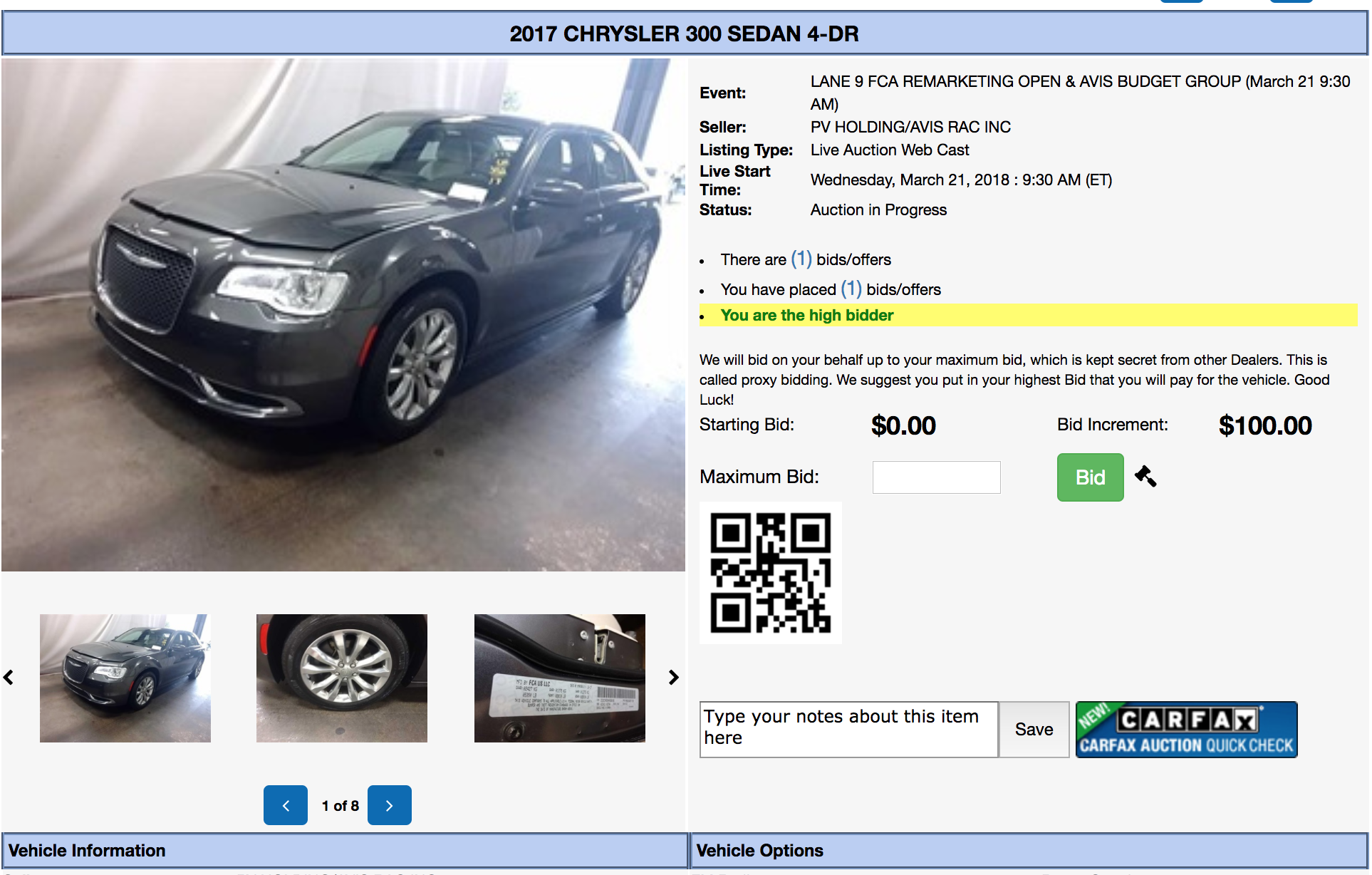This image depicts a webpage dedicated to vehicle trade-ins, focusing primarily on a 2017 Chrysler 300 sedan. The top of the webpage features a blue banner with bold, black lettering, drawing attention to the site's purpose. Below this banner, the page is divided into two main sections. 

The left half showcases an eye-catching photograph of the Chrysler 300, allowing viewers to examine the car's exterior. Its sleek design and metallic finish are prominently displayed, indicating it's well-maintained and appealing to potential bidders.

The right half of the image is a detailed information panel. Here, users can find comprehensive details about the vehicle, including specific auction information such as the date, location, and various bidding options available. This section ensures that interested buyers have all the necessary information at their fingertips.

At the bottom of the page, another blue banner with the headings "Vehicle Information" and "Vehicle Options" offers further insights into the car's features and capabilities, rounding out a full, informative presentation meant to assist potential buyers in making an informed decision.